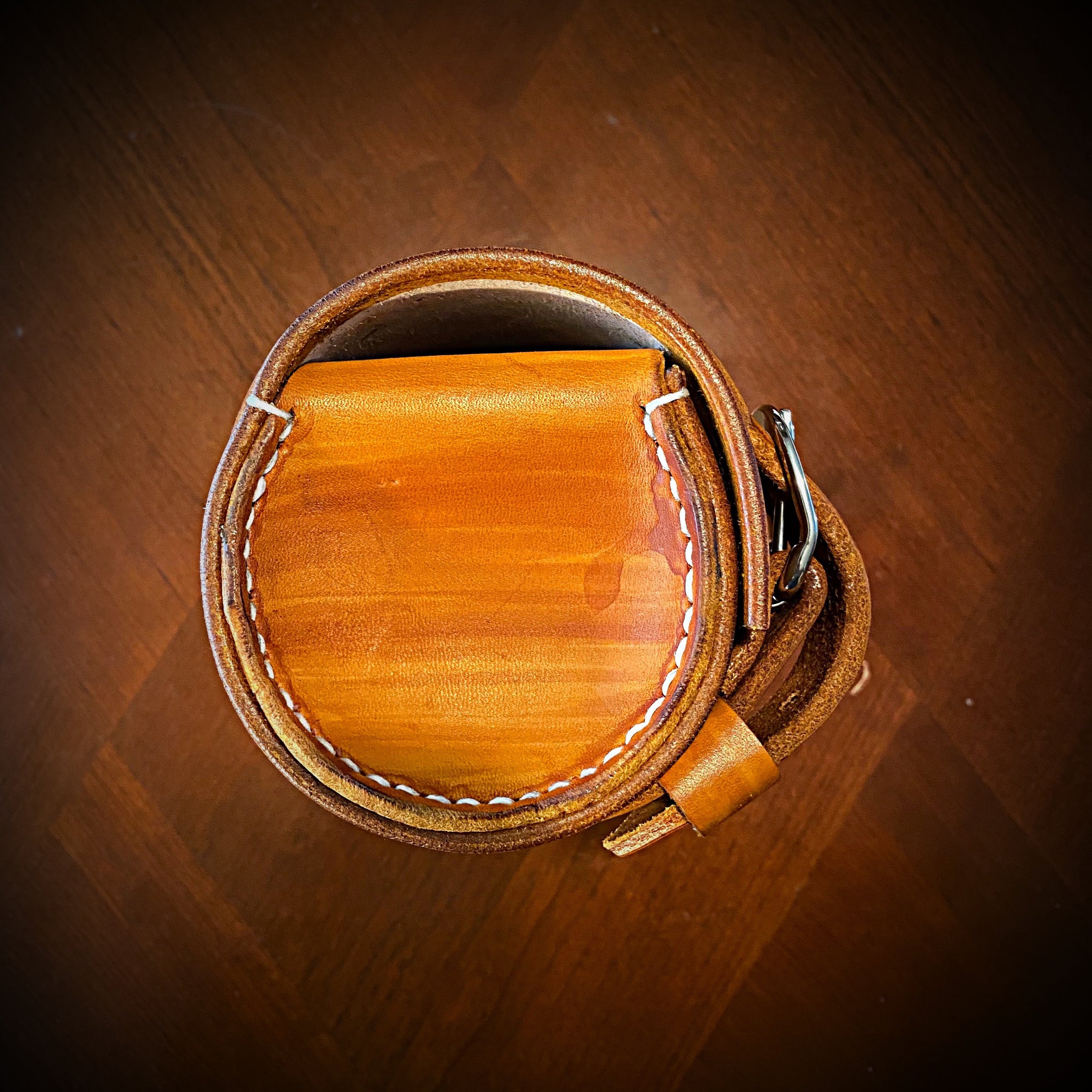The image is a near-square, slightly taller than wide, featuring a richly textured brown background with diagonal lines descending from the top left and a subtle square within the square at the bottom, resembling a diamond shape. Central to the image is a detailed portrayal of a leather accessory, which appears to be a hybrid between a belt and a pouch, designed to be worn around the waist. The main compartment of the pouch is a yellowish-brown color with light striping and a textured finish, adorned with white stitching in a U-shape around its bottom. The object includes a prominent leather belt-like strap, also brown, secured on the right side with a silver buckle. The entire piece, potentially resembling a small holster, rests on what seems to be a dark red-brown hardwood floor, possibly parquet style, adding contrast and enriching the overall aesthetic of the image.